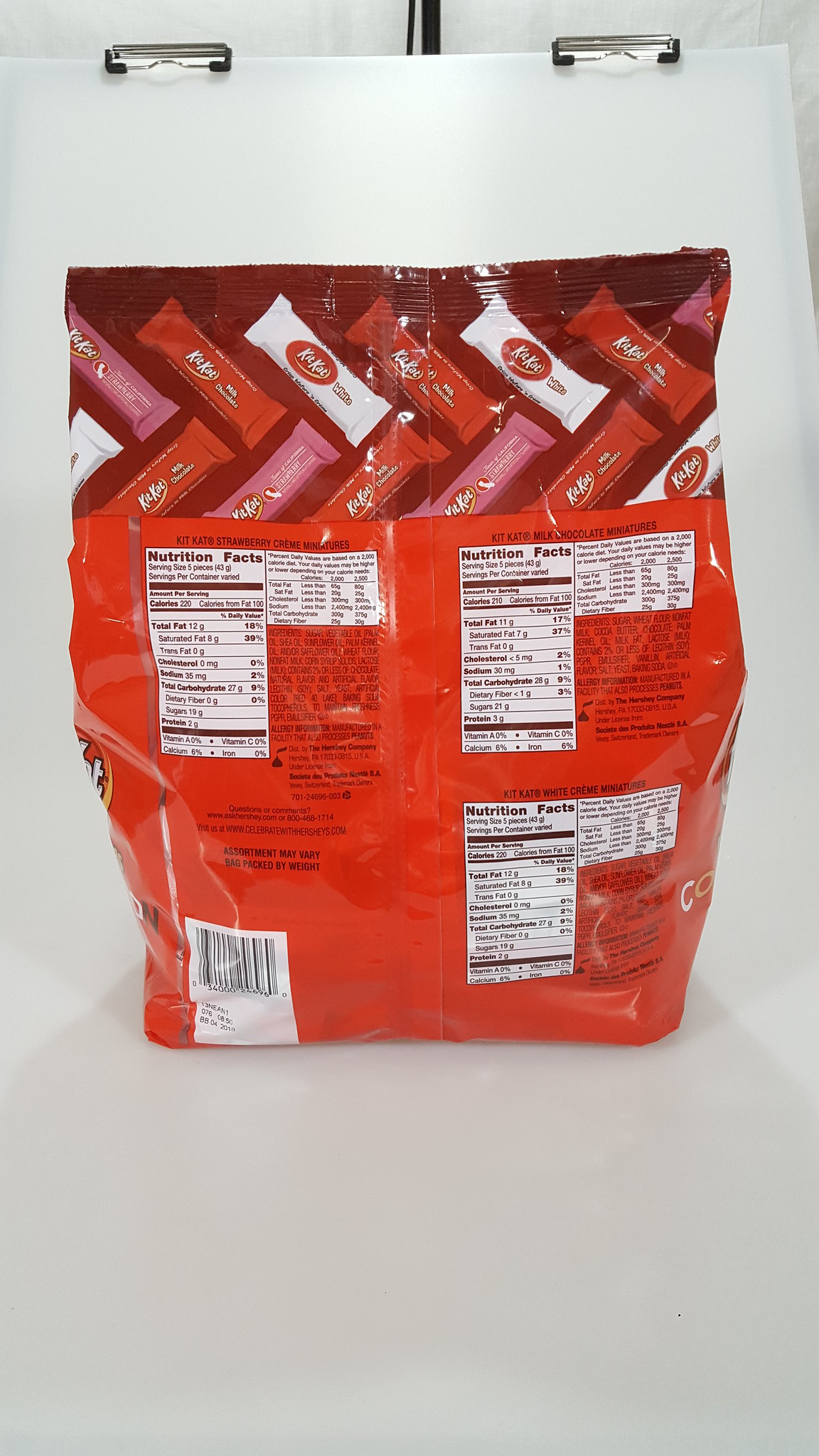This is a photograph of the back of a large KitKat bag, displayed against a white background that's held up by two black metal clips at the top. The bag itself is prominently featured in the center. The top section of the bag displays various small, individually wrapped KitKat bars in different colors and styles, including white, purple, red, and green. Below this colorful display, the background of the bag turns red and showcases three separate Nutrition Facts labels, each accompanied by its own ingredients list. At the bottom left corner of the bag, a barcode is set against a white background. The sides of the bag feature larger KitKat logos, and the entire bag has a white backdrop, throwing a noticeable shadow on the surface below.